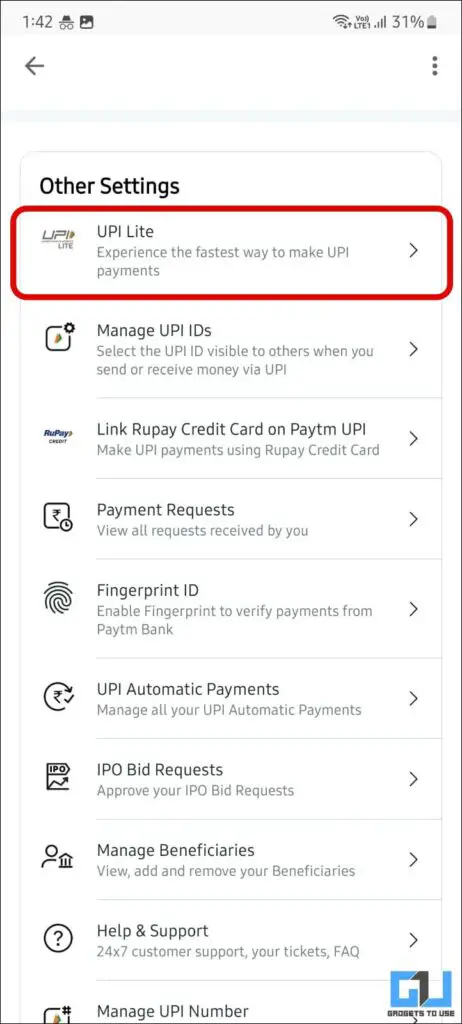This image is a screenshot of a cell phone display captured at 1:42 AM or PM (time not specified). The phone indicates an active Wi-Fi connection, a cell signal, and a battery charge of 31%, visible in the upper right corner of the screen. Just below this, there is a navigation bar with a back button on the left and a menu icon represented by three vertical dots on the right.

The main content of the screenshot focuses on the section titled "Other Settings." The first option, highlighted with a red rectangle, is "UPI Lite," promoting itself as the fastest way to make UPI payments and includes a right-pointing arrow for further interaction. Following this are several other options presented with right-facing arrows:

1. **Manage UPI IDs:** Allows users to select which UPI ID is visible to others when sending and receiving money via UPI.
2. **Link RootPay Credit Card on PayTM UPI:** Provides the ability to make UPI payments using the RootPay credit card.
3. **Payment Request:** Enables the user to view all payment requests received.
4. **Fingerprint ID:** Allows enabling fingerprint verification for payments.
5. **UPI Automatic Payments:** Lets users manage all their UPI automatic payments.
6. **IPO Bid Requests:** Offers approval options for IPO bid requests.
7. **Manage Beneficiaries:** Presumably for managing the users' list of beneficiaries.

Each feature is detailed with a summary of its function, ensuring comprehensive control over various UPI payment options and settings.